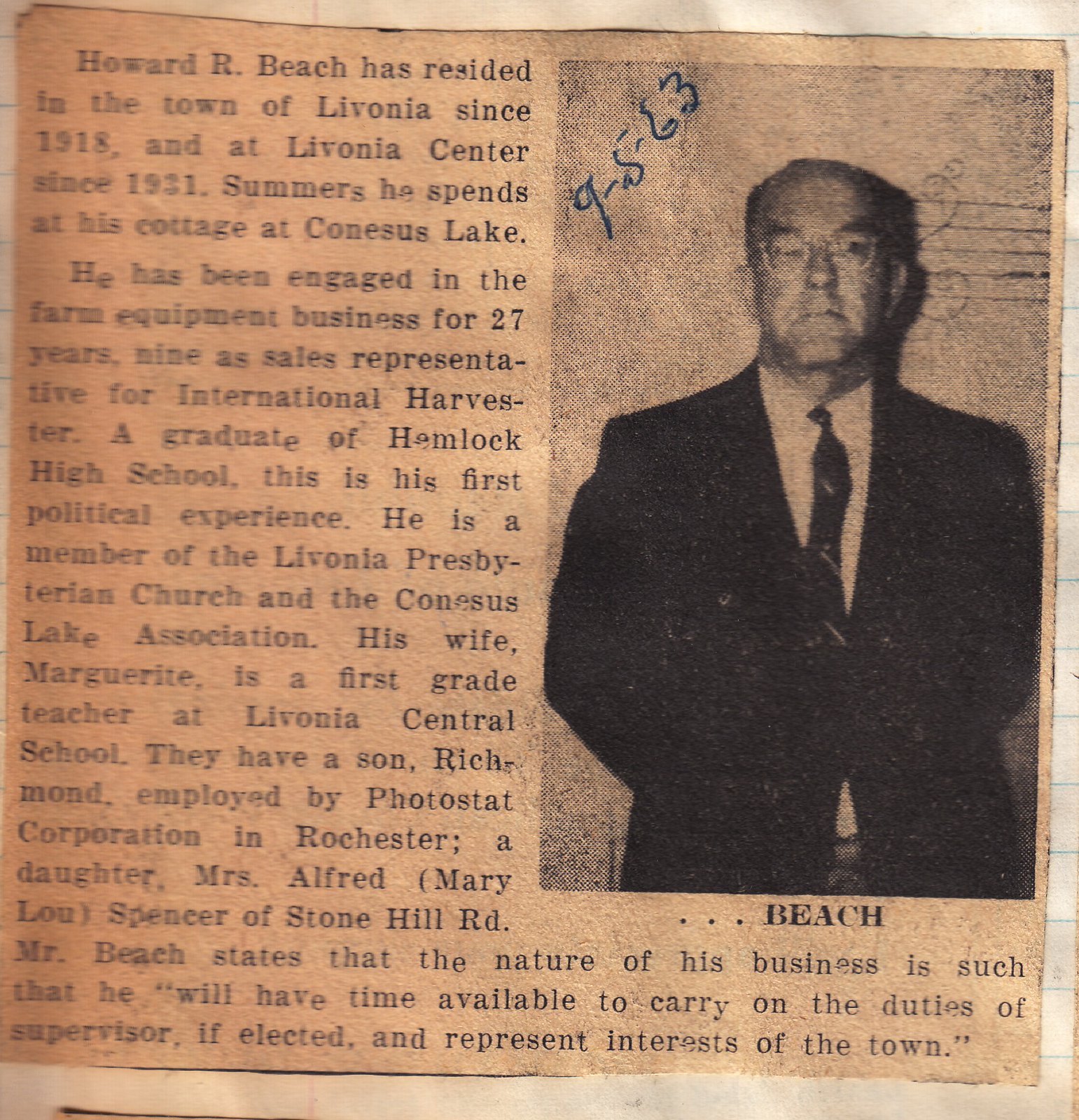This image features a sepia-toned, aged newspaper clipping pasted onto notebook paper, with handwritten blue ink that reads "9-5-63" at the top left corner. The clipping includes a black and white photograph of an older man in a suit, labeled "Beach" beneath it. The article details Howard R. Beach's life and achievements, stating that he has resided in the town of Livonia since 1918 and at Livonia Center since 1931. During summers, he spends time at his cottage at Conesus Lake. With 27 years of experience in the farm equipment business, including nine as a sales representative for International Harvester, this is his first venture into politics. A Hemlock High School graduate, Beach is involved with the Livonia Presbyterian Church and the Conesus Lake Association. His wife, Marguerite, teaches first grade at Livonia Central High School. They have two children—Richard, who works for Photostat Corporation in Rochester, and Mrs. Alfred Mary Lou Spencer, who lives on Stonehill Road. Howard Beach commits to dedicating ample time to his duties as a supervisor if elected, ensuring representation of the town's interests.